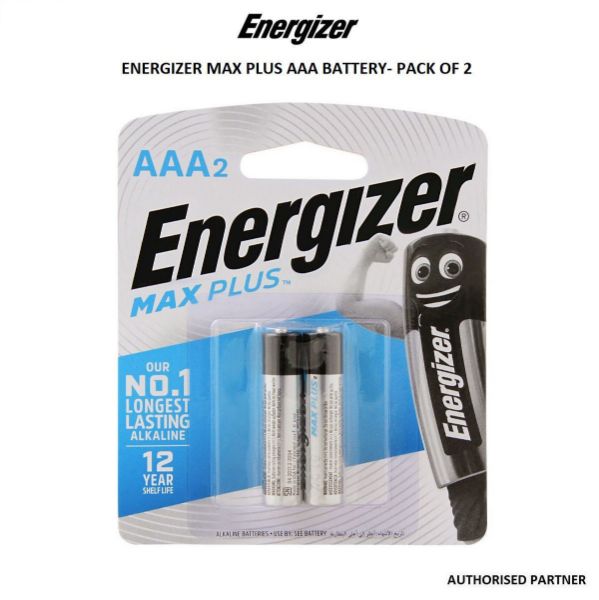This is a detailed screenshot of an Energizer battery product. At the top of the image, the brand name "Energizer" is prominently displayed in bold black italic letters. Underneath this, in smaller text, it reads "Energizer Max Plus AAA Batteries - Pack of Two." 

The central portion of the image features a clear stock photo of the item itself—two AAA Energizer Max Plus batteries encased in plastic packaging. The packaging has a white background adorned with black spiral designs. In the top left corner, the label "AAA2" is highlighted in blue.

To the right of the batteries, there’s a whimsical graphic depicting an Energizer battery with human features, smiling broadly and flexing its arm muscle in a show of strength. To the left, text boasts "Our #1 Longest Lasting Alkaline - 12-Year Shelf Life."

Below the batteries, fine print text reads "Alkaline Batteries - Use By," followed by an expiration date. At the bottom right corner of the image, just outside the packaging, there is a label that reads "Authorized Partner," adding an element of authenticity and trust.